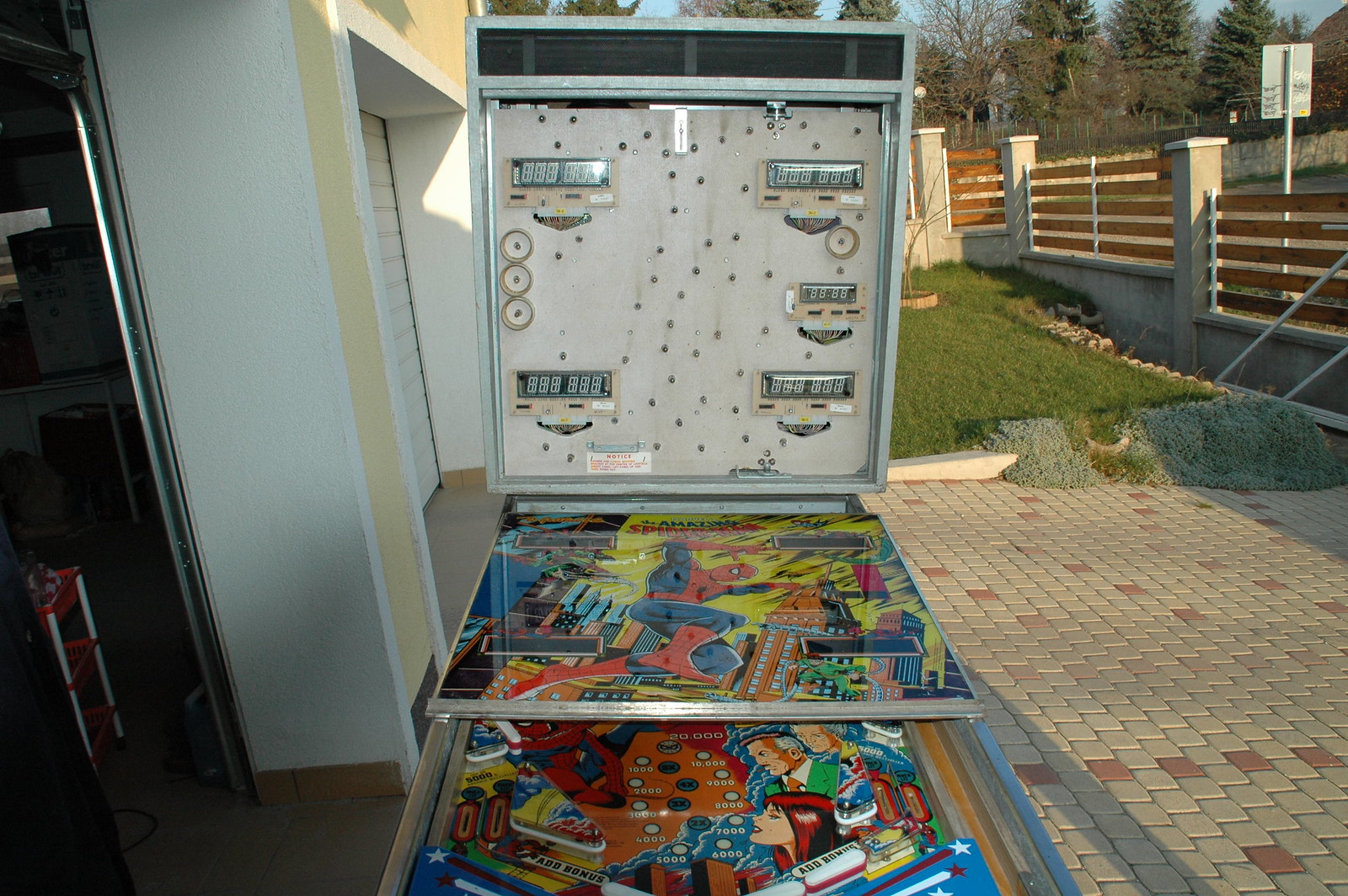This photograph captures a discarded Superman-themed pinball machine situated outdoors, possibly in a driveway or a patio area that appears to be part of a public storage facility or someone's property. The backdrop features whitewashed walls, a garage door on the left, and a stone patio with brick tiles in beige and red hues. The machine itself is positioned with its glass cover open, revealing digital knobs and score displays. The levers, typically used to control the game's flippers, are visible along with the intricate, colorful designs associated with a Superman theme. Surrounding the area, there's a wooden fence with a concrete base and concrete pillars, flanked by some trees, adding a sense of enclosure and seclusion to the setting. The scene is further characterized by the mixed architectural elements like an incline that leads to a gate, emphasizing the storage or transitional nature of the location.